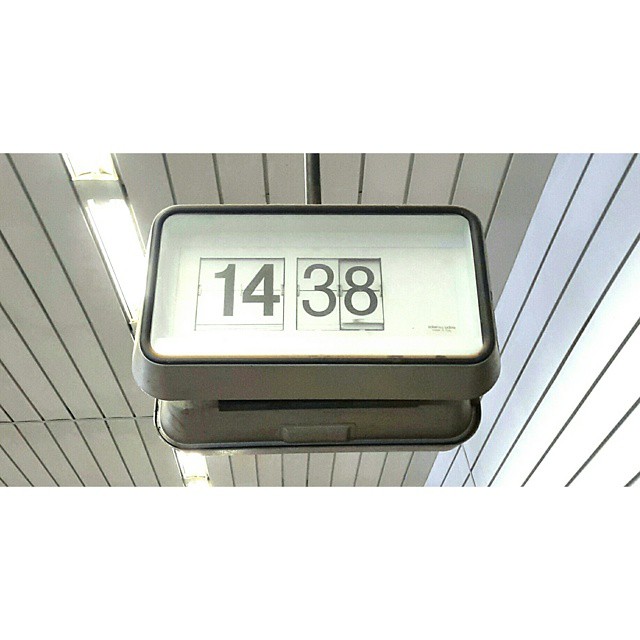The image depicts a digital clock hanging from a white slatted wooden ceiling, viewed from below. The clock, housed in a black square case with a prominent black bar securing it to the ceiling, displays the time "14:38" in bold black digital numbers on a white face. The ceiling, covered with white planks lined with grout, creates a structured backdrop, and features narrow iridescent lights running along the left side, contributing to a reflective, elongated visual effect due to mirrored surfaces beneath. The clock, with numbers organized in distinct boxes—thicker for the hour and thinner for the minutes—suggests a functional setting, reminiscent of places like hallways in offices, retail stores, airports, or possibly a train station, where utilitarian design and clear visibility are paramount.